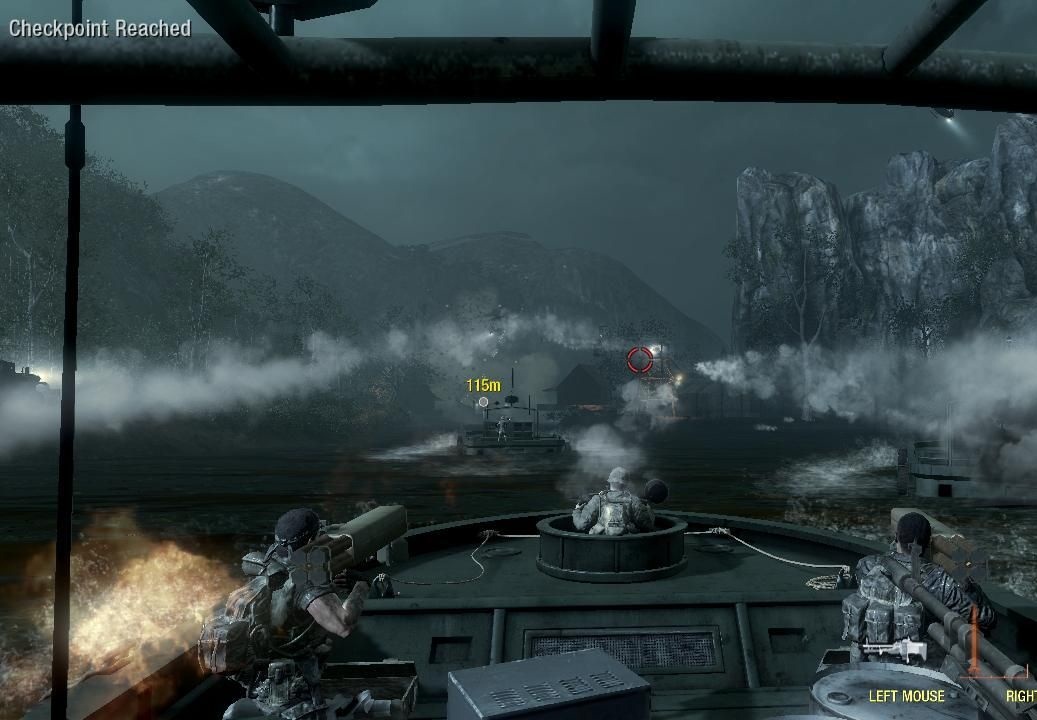The image appears to be a screenshot from a video game. The player, positioned on a raised deck, overlooks a scene featuring numerous graves. In the foreground, military personnel clad in protective gear, including helmets, are visible manning a military vehicle that resembles a boat, tank, or carrier. The player’s heads-up display (HUD) indicates controls labeled "left mounts" and "right," with a distance marker showing "115 meters." The setting includes a road flanked by fog on either side, while distant mountains frame the scene, extending into the horizon.